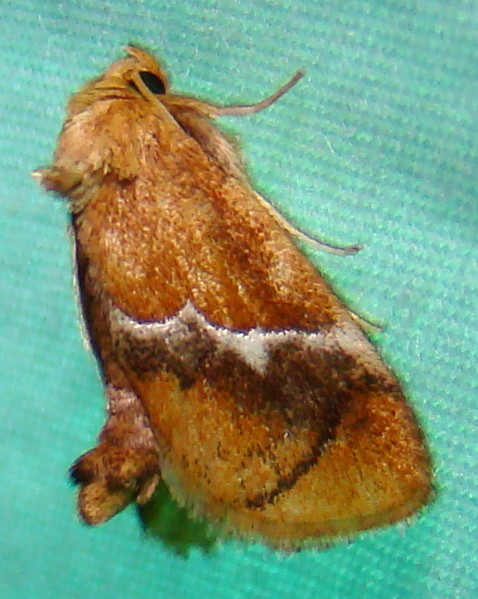In the image, a hairy moth is depicted resting on a lightish green, bubble-textured background that might resemble turquoise or teal cloth. The moth's side-facing view showcases its oval, teardrop-shaped wing, which is predominantly golden brown with a jagged white stripe cutting across the middle. Above the stripe, there is a darker brown section, while the lower part remains a lighter brown. Thin legs extend from the moth’s front, leading to a hairier neck area. The head is discernible, featuring a prominent black eye. At the top of the wing, white string-like structures are visible, and towards the back, the moth's body is faintly outlined.